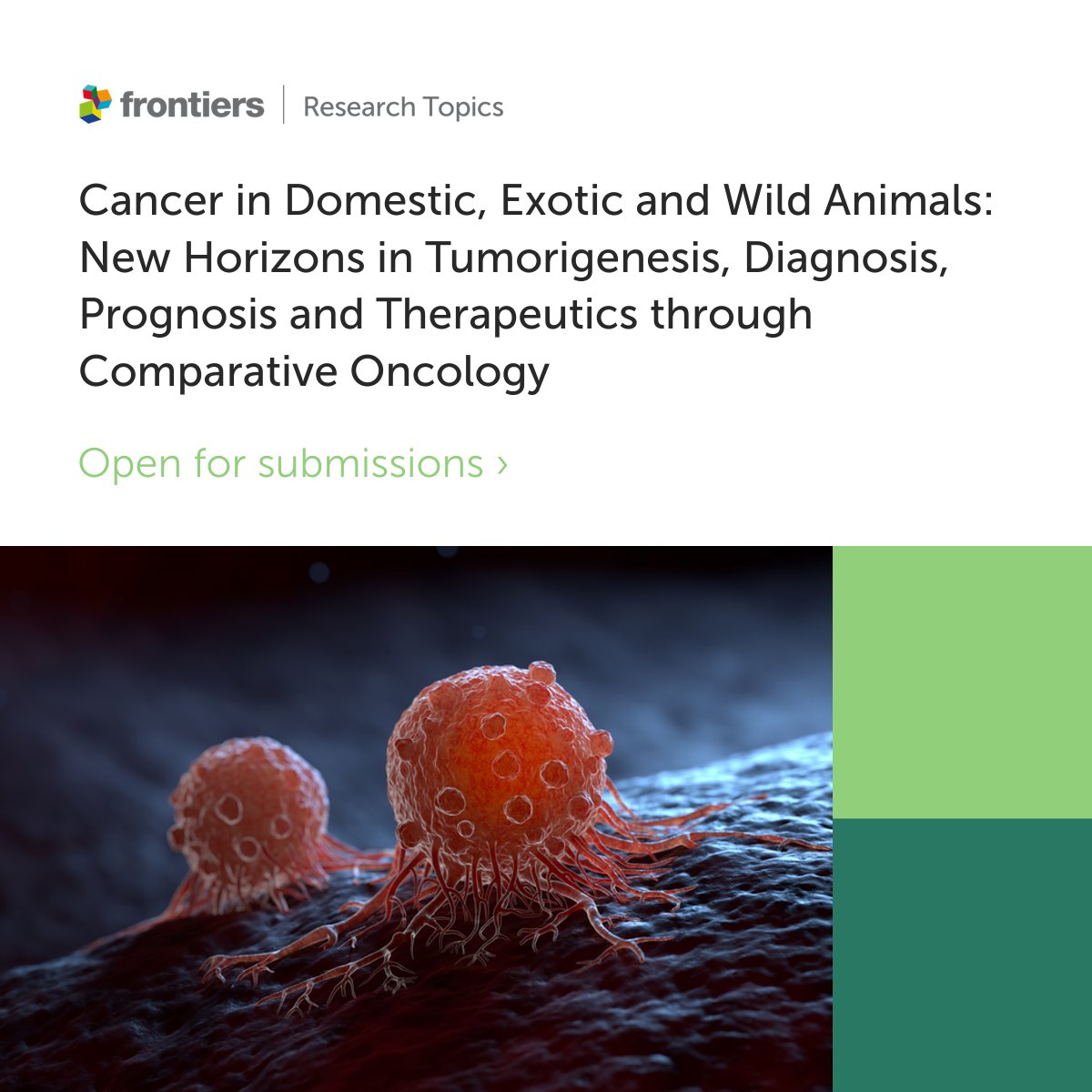The image is a highly detailed, horizontal illustration resembling a microscopic view, possibly using a Scanning Electron Microscope (SEM) technique, depicting two spherical, red lumpy bacteria or cancer cells with tentacle-like extensions grabbing onto what appears to be human skin or stroma. The cells are attempting to establish themselves in the host. On the right side of the image, there are two homogeneous light green and light blue squares. This artwork is featured in a call for papers from the journal "Frontiers," focusing on cancer in domestic, exotic, and wild animals, and highlights new horizons in tumor genesis, diagnosis, prognosis, and therapeutics through comparative oncology.